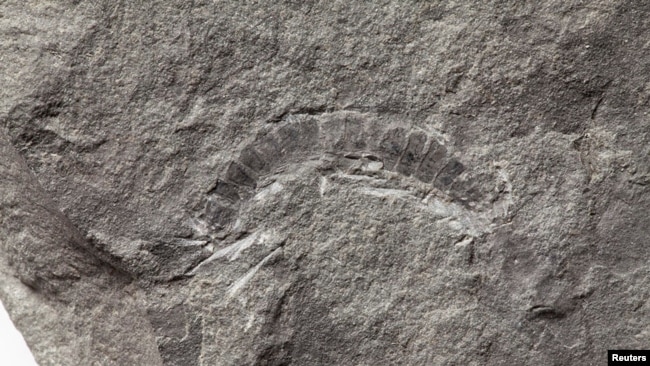The image features a detailed fossil embedded in a grey and whitish rock, possibly granite. The fossil, situated centrally, has a curvy, segmented shape that resembles a worm but could be interpreted as an insect, reptile, snake, or caterpillar. The rock surface is predominantly grey and white, enhancing the fossil's intricate patterns. At the bottom right corner of the image, the word "Reuters" is inscribed in white against a black background.